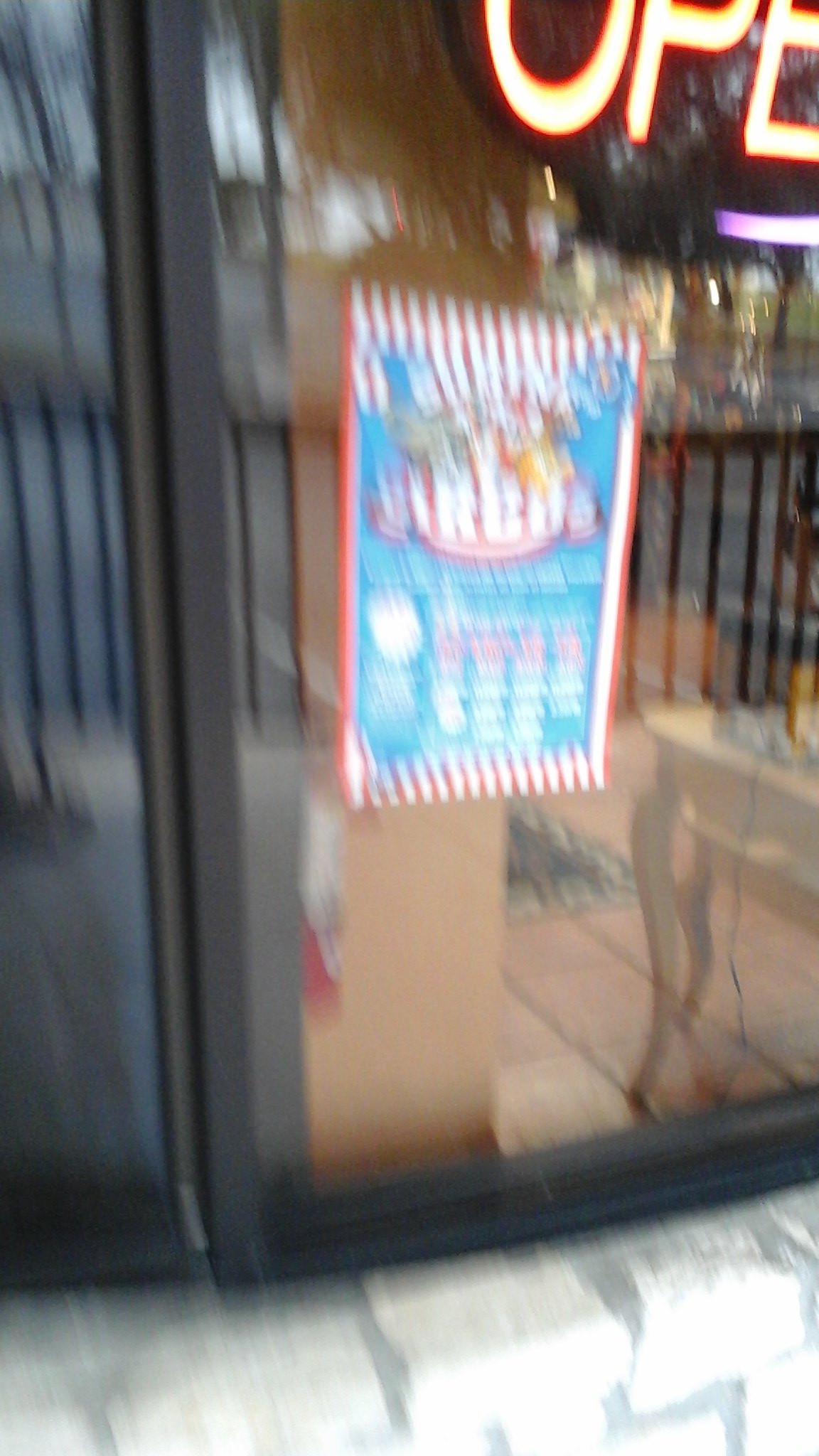A photograph captures the exterior of what appears to be a restaurant or a store, illuminated by a neon "OPEN" sign. The sign is only partially visible, showing the letters "O," "P," and "E" in the top right corner and a glowing purple swirl that extends to the bottom right of the sign. Below this sign, centrally positioned, hangs a vibrant poster promoting a circus. Despite the blurriness of the image—likely due to the photographer's motion—details of the poster emerge. It features the word "CIRCUS" prominently, partially visible through the blur. The poster's design includes a red outline with white stripes along the top, bottom, and right edges. In the blue background, faint shapes suggest the presence of circus animals near the logo. The overall scene is vivid yet marred by the motion-induced blur, creating a dynamic yet unclear visual narrative.